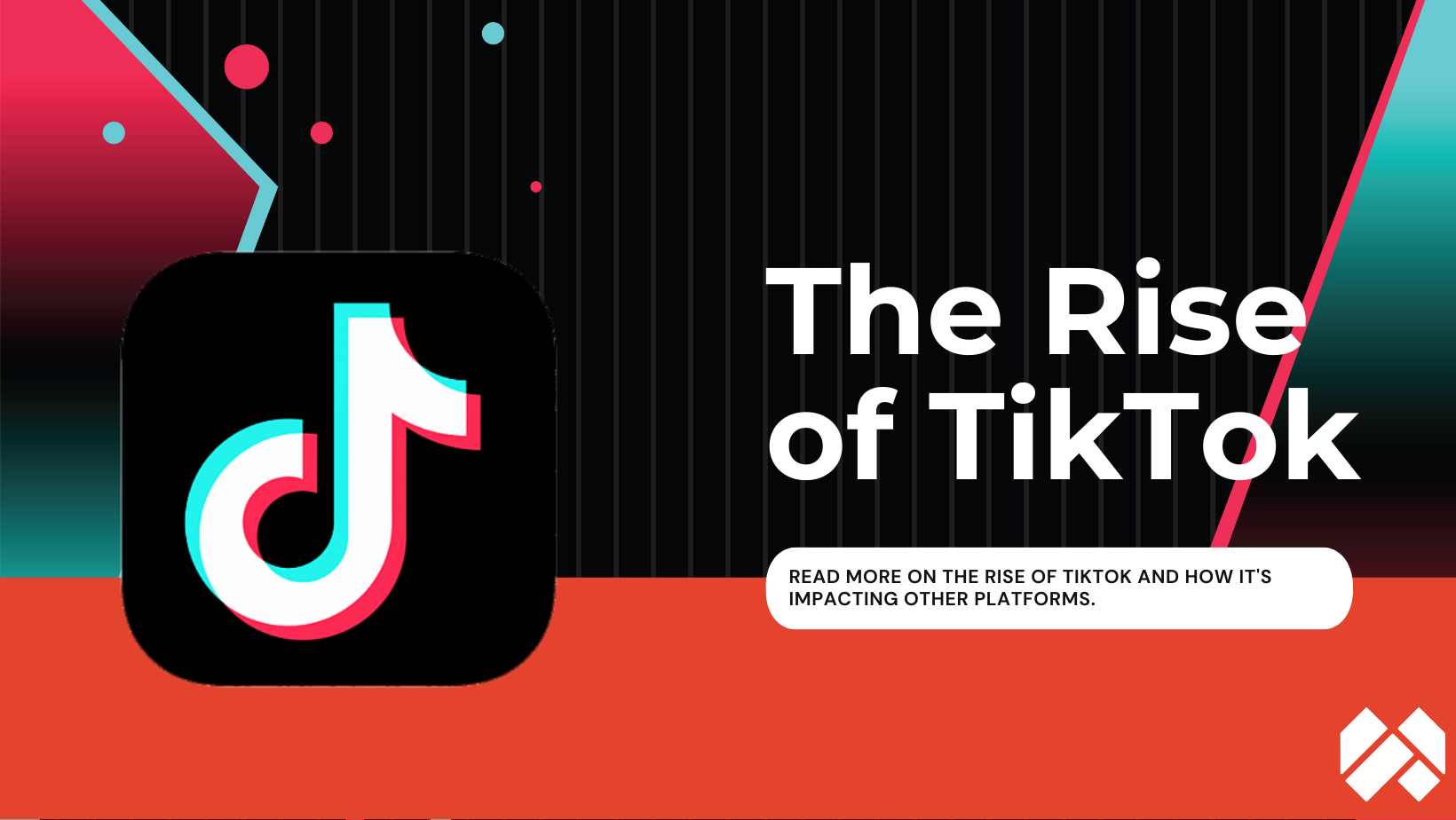In this vibrant image, a large title "The Rise of TikTok" is prominently displayed in bold, white text, capturing the viewer's attention immediately. The TikTok logo, resembling a stylized musical note with a playful and intriguing design, accompanies the title. Just below the main text, within a white bubble featuring black text, an invitation to "Read more on The Rise of TikTok and how it's impacting other platforms" is clearly visible.

The background of the image is primarily a vivid red, enriched by gradients of forest green and punctuated with a scattering of aqua blue-green and red dots. Adding to the visual complexity, there is a distinctive white symbol located in the bottom right-hand corner, complementing the overall composition.